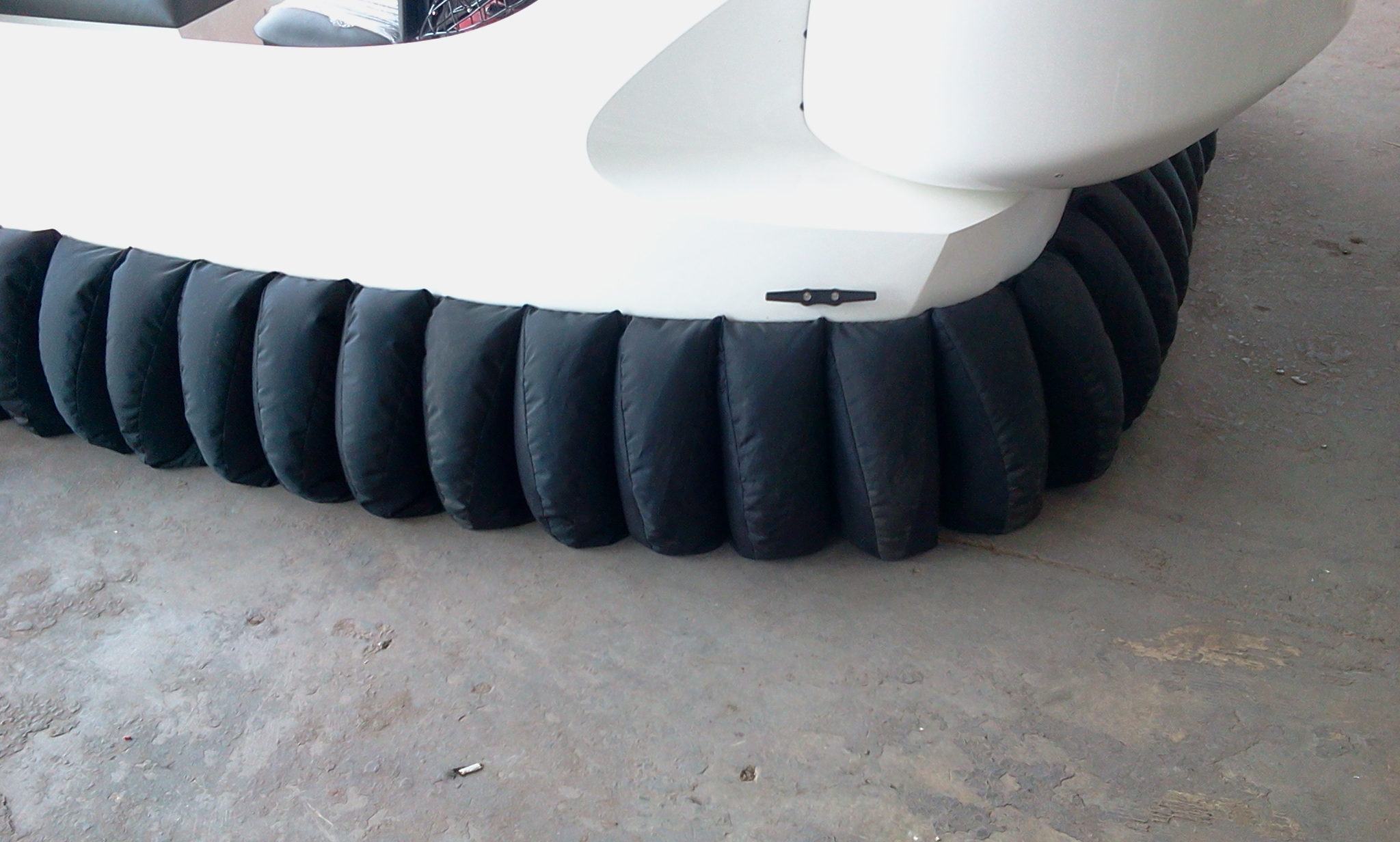This color photograph captures a mysterious object partially cropped at the top, resting on a weathered, gray concrete floor marked with slight orangish-yellow discolorations. The object features a black, cushion-like base with evenly spaced, soft protrusions, giving it the appearance of an inflatable structure such as an airbag or air mattress. Above the black base, the object transitions into a smooth, white section, possibly made from a futuristic, plastic-like material. This upper white portion might include an indentation, hinting at potential storage for chairs or other items. Notably, a stubbed-out cigarette butt can be seen on the concrete floor near the bottom center of the image. The photograph excludes any visible writing, people, or animals, emphasizing the enigmatic nature of the scene.